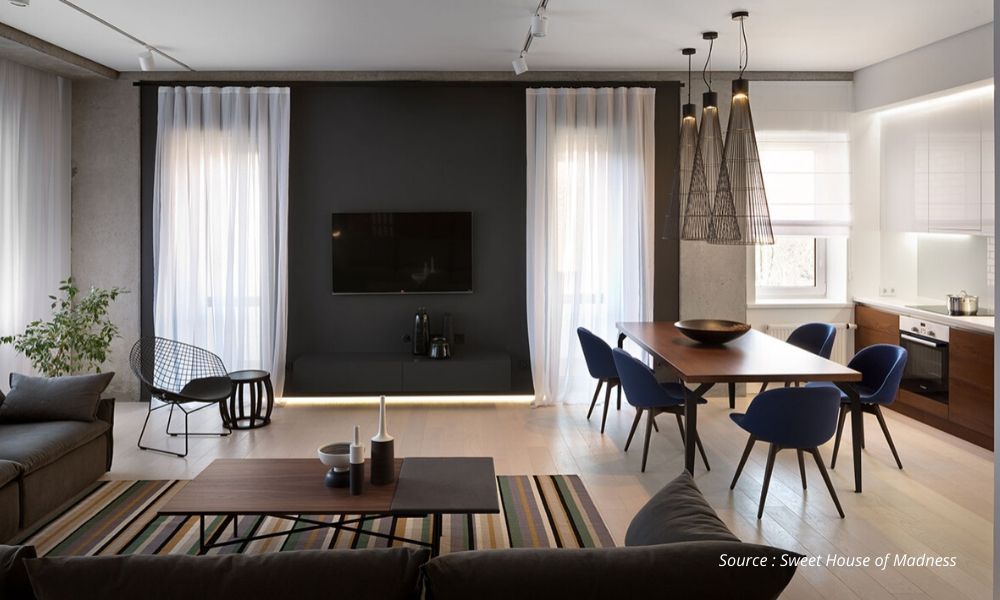This photograph captures a beautifully designed open-concept living area, characterized by its harmonious blend of browns, grays, whites, and subtle blue accents. The image is taken from behind an L-shaped upholstered couch, which features matching throw pillows that enhance its inviting appearance. In front of the couch lies a tan, brown, gray, and white striped rug that complements the space's earthy tones. Atop the rug sits a low wooden coffee table with ornate wrought iron legs, adorned with three pottery decorative elements in shades of white, blue, and brown.

The far wall is dominated by a gray hearth fireplace with a sleek, modern TV mounted above it, flanked by floor-to-ceiling sheer white curtains that add a touch of elegance. In front of the fireplace, a wire mesh chair accompanied by a wooden ottoman offers a cozy nook for relaxation. To the right, a long Danish-style wooden table is surrounded by five mid-century modern dining chairs upholstered in a rich blue fabric. A striking round brass bowl serves as the centerpiece on this stylish table.

Further right, the kitchen seamlessly integrates with the living space. It features lower brown cabinetry with a built-in oven and a cooktop, on which a silver soup pot rests, ready for the next culinary creation. This thoughtfully designed interior embodies a perfect balance of comfort, style, and functionality.